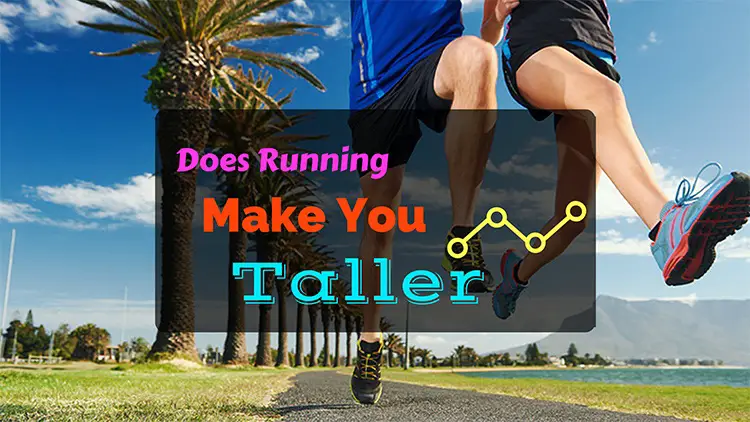The vibrant photograph captures the lower halves of two runners, actively sprinting along a semi-paved path near a serene lake, framed by a backdrop of lush palm trees, a bright blue sky, and distant mountains. The runners, visible from just below their stomachs to their feet, showcase a dynamic stride with one runner donning black sneakers and the other sporting light blue and red sneakers. Above the vivid scene, a black translucent rectangle features the text, "Does running make you taller?" The words are colorfully segmented with "does running" in magenta, "make you" in red, and "taller" in turquoise, and accompanied by a yellow zigzag line design composed of circles and connecting lines. The picturesque tropical setting enhances the energetic ambiance, suggesting an advertisement for either shoes or exercise, evoking thoughts about the potential benefits of running.